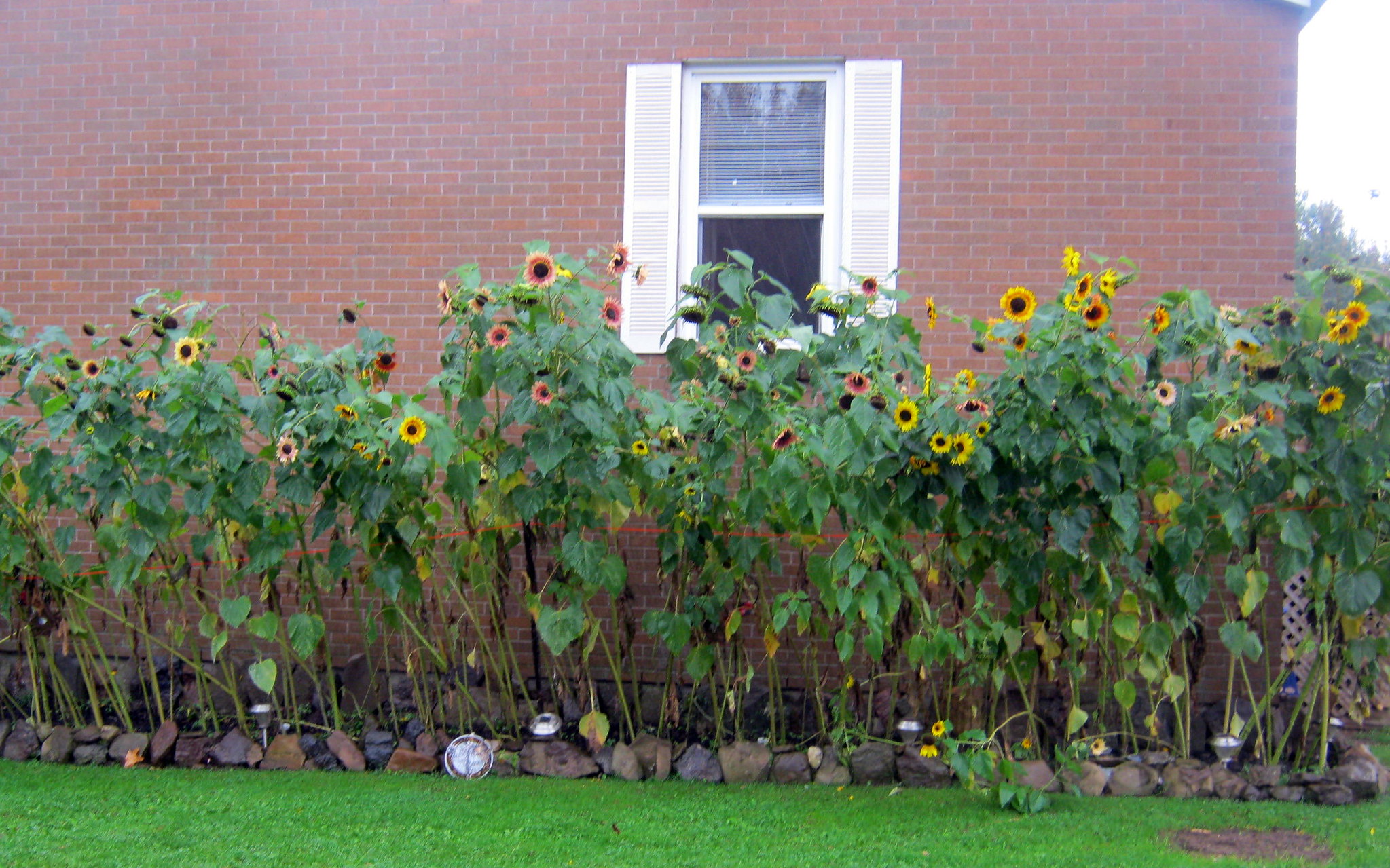The photograph captures a vibrant garden scene beside a traditional red brick house. Dominating the right side of the image is the house itself, with a singular white-framed window adorned with white shutters and partially open white mini blinds. Spanning nearly the entire length of the house is a meticulously maintained flowerbed, bursting with tall sunflowers and a few pink-hued varieties, their brilliant yellow petals encircling rich brown and black centers. In front of the flowerbed lies a well-manicured green lawn, interrupted only by a small patch of dirt in the bottom right corner. The scene is bathed in natural light, with a bright blue sky peeking through at the top right, adding to the garden's lively atmosphere. A small stone path runs along the garden bed, providing a neat division between the lush greenery and the house.